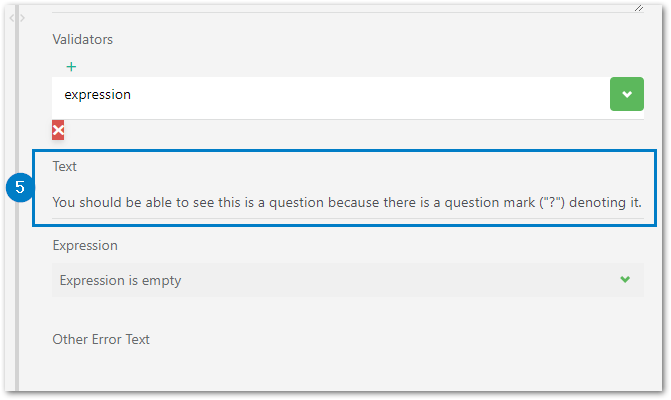A cropped screenshot, likely taken from a website or computer software application, features a light grey background. At the top, there's a title labeled “Validators.” Directly beneath this title is a green drop-down arrow with the word “Expression” displayed inside the drop-down box. Just below, a small red rectangle with a white "X" inside is present. Further down, a block of text reads: "You should be able to see this is a question because there is a question mark denoting it," encased within a blue highlighted rectangle with the number "5" adjacent to it. Below this highlighted section, another section titled "Expression" appears, featuring a drop-down box with the text "Expression is empty." At the very bottom of the screenshot, the words "Other error text" are visible. The absence of additional details or elements makes it difficult to ascertain the full context of the image.